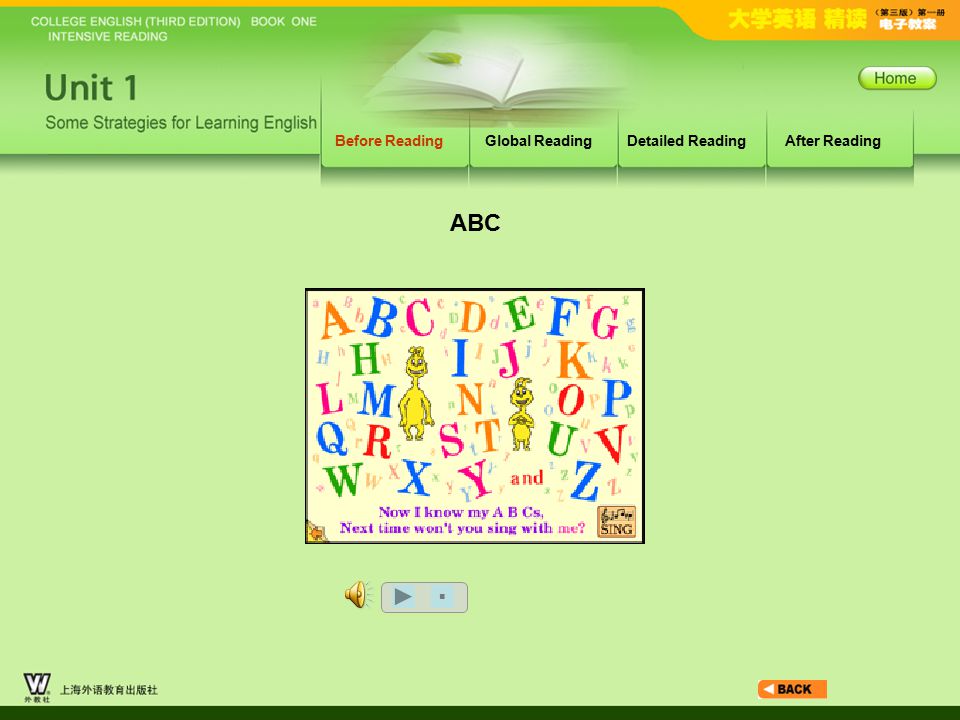The image showcases a vibrant and educational web page set against a green background with a darker green header. The header features white text on the upper left, stating, "College English, 3rd Edition, Book 1, Intensive Reading." At the center of this header is an illustration of an open white book. In the upper right corner, there is a small orange banner adorned with Asian characters. Below this banner, on the left side, it reads, "Unit 1, Some Strategies for Learning English."

To the right, there are several red and black menu buttons: "Before Reading" in red, and "Global Reading," "Detailed Reading," and "After Reading" in black. A green "Home" button is located in the upper right corner of the page.

Further down, against a lighter green background, a black-outlined white box displays a colorful array of alphabet letters in shades of blue, purple, orange, and red. In the center of this box, two whimsical characters reminiscent of Dr. Seuss's illustrations are prominently featured. Below this illustration, the text reads, "Now I Know My ABCs, Next Time Won't You Sing With Me?" adding a playful and musical element to the page.